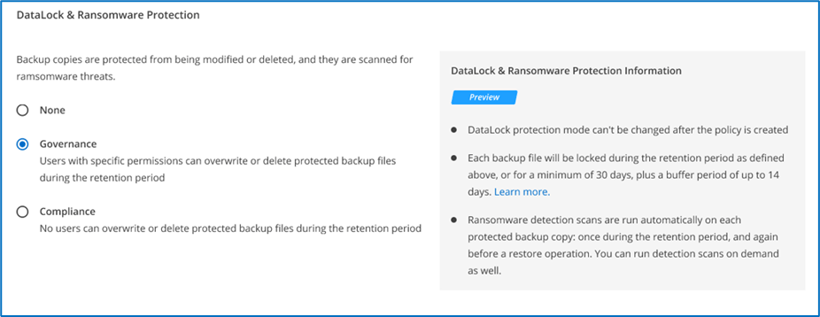**Detailed Caption:**

The image is a horizontally oriented web graphic set against a white background and bordered by a thin blue outline. Positioned in the upper left-hand corner is the header "Datalog and Ransomware Protection." Beneath this, the text states: "Backup copies are protected from being modified or deleted and they are scanned for ransomware threats."

Below the introductory text are three selection boxes accompanied by circles to their left, marked as None, Governance, and Compliance. The Governance option has been selected. For the Governance option, the description reads: "Users with specific permissions can overwrite or delete protected backup files during the retention period." Retention period specifics for the Compliance option state: "No users can overwrite or delete protected backup files during the retention period."

Adjacent to these options, on the right side of the image, is a very light gray box titled "Datalog and Ransomware Protection Information." Underneath this title is a button labeled "Preview." The gray box lists three vertical bullet points detailing further information:

1. "Datalog Protection Mode can't be changed after the policy is created. Each backup file will be locked during the retention period as defined above or for a minimum of 30 days plus a buffer period of up to 14 days. [Learn More]"
2. "Ransomware detection scans are run automatically on each protected backup copy once during the retention period and again before a restore operation."
3. "You can run detection scans on demand as well."

These bullet points provide additional context and governance specifics regarding the functionality and policies for datalog and ransomware protection.